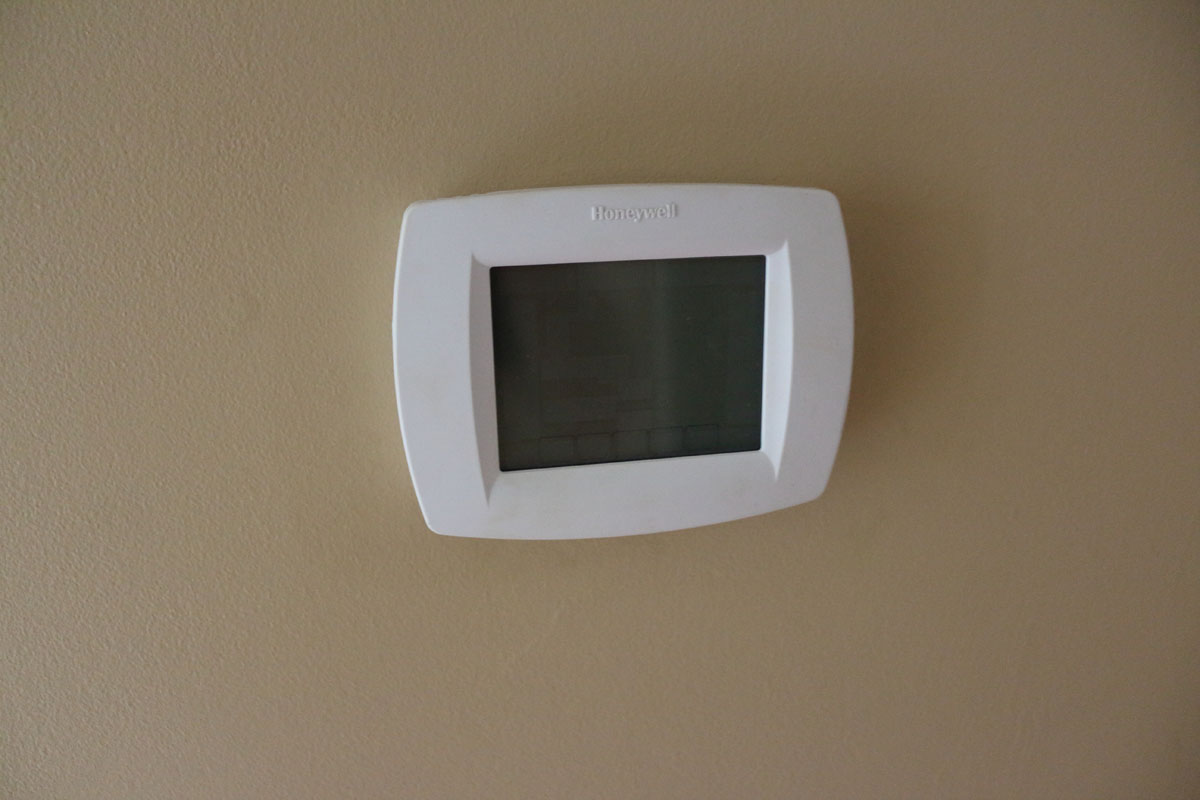The image depicts a tan wall uniformly shaded with a lack of any significant definition or texture, except for a subtle interplay of shadows. Mounted centrally on this smooth wall is a white plastic frame encasing a gray plastic center. This central object is a Honeywell thermostat. Although the text and markings in dark lettering beneath the gray center are present, they are not illuminated, rendering them unreadable. The top of the thermostat features the brand name "Honeywell" embossed in the center. A faint gray shadow appears above the thermostat, while a darker shadow falls to the right side, suggesting that the light source is positioned to the left, casting pronounced shadows to the right of the thermostat.